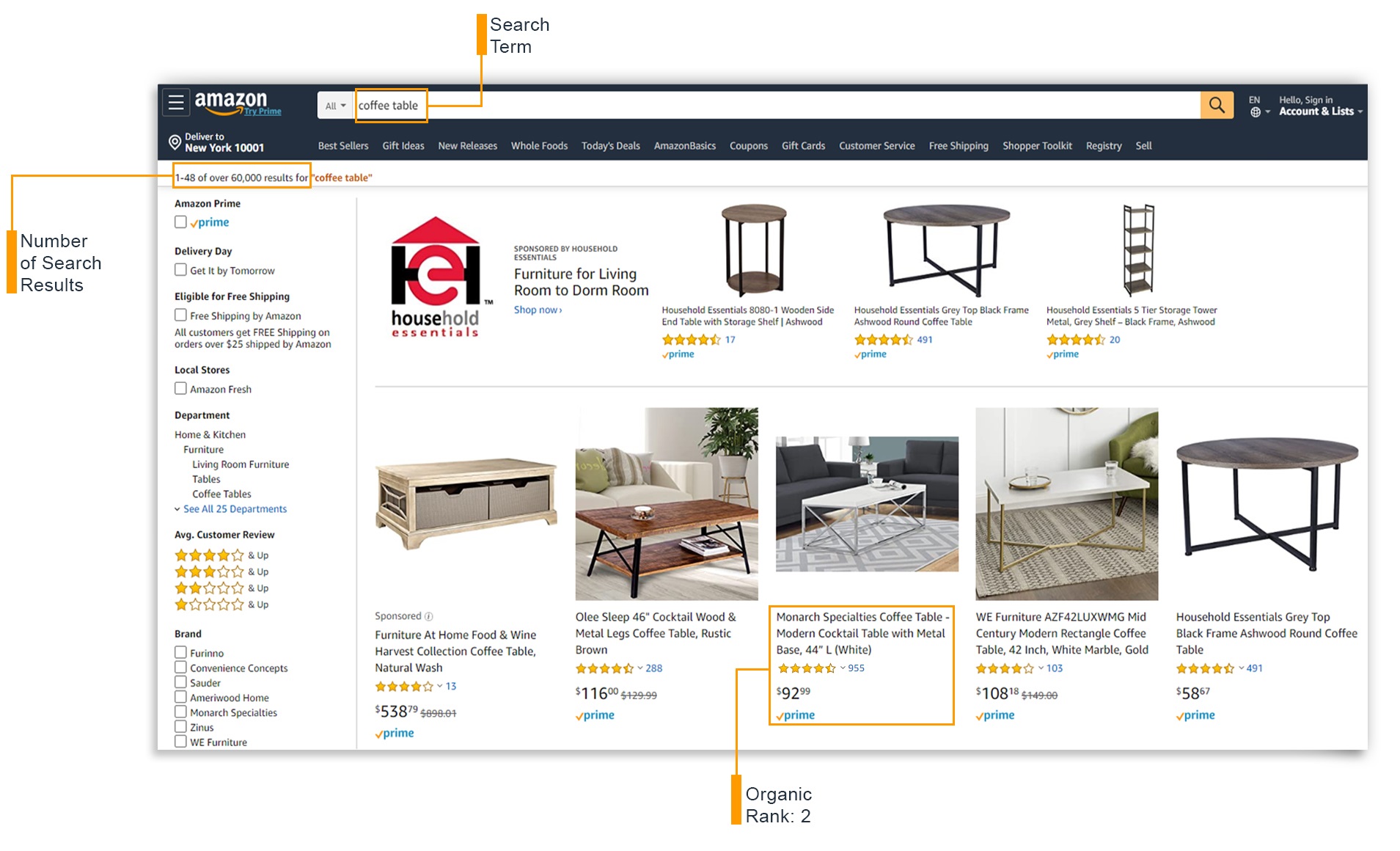Here is a cleaned-up and more detailed caption for the image:

---

The webpage displayed is a search results page for "coffee table" on Amazon.com. At the top, the search bar shows the user's query for coffee tables. On the left side of the page, there are filters for customer review ratings and selectable brands. The search results summary is highlighted with a yellow square, indicating "1-48 of over 60,000 results for coffee table."

Below the search summary, various coffee tables are displayed with corresponding advertisements. In the top section, there's a sponsored advertisement by Household Essentials featuring their logo "HE" in the middle and three distinct coffee tables to the right of it.

Directly beneath this ad, there are five additional coffee tables listed as search results. The third table in this list is surrounded by a yellow square — signifying it’s highlighted and marked as "Organic Rank #2," though the significance of this ranking isn't clear. The highlighted table is a white coffee table priced at $92.99. Unlike the first table, which is labeled as sponsored, this table and the other four in its section are not marked as sponsored ads.

---

This enhanced description captures the primary elements of the webpage, adding clarity and coherence to the given content.